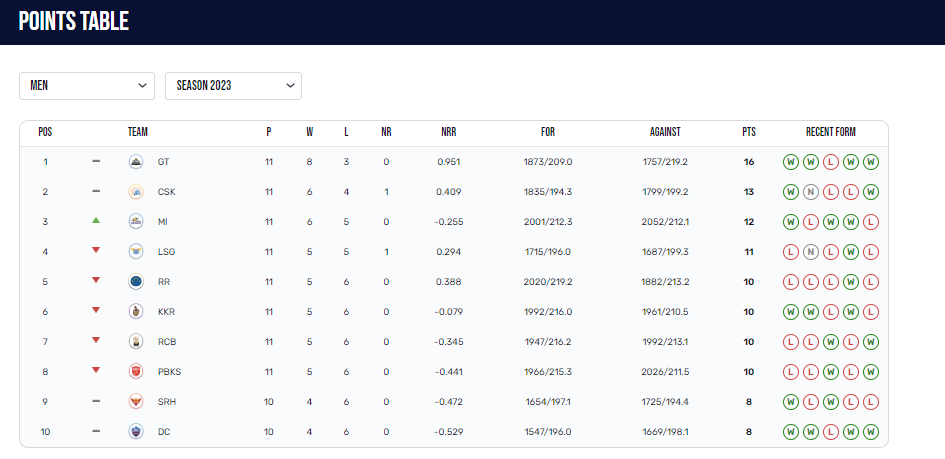Screenshot of the Points Table for the 2023 Men's Sports League

The page header showcases a black or dark blue background with the prominent all-caps white text "POINTS TABLE" positioned in the upper left corner. Directly beneath the header, there are two sorting boxes. The first box is labeled "MEN" in all caps, accompanied by a right-pointing drop-down arrow. Adjacent to this is another box labeled "SEASON 2023," also in all caps, with a similar drop-down arrow.

The table itself is neatly outlined with a light gray border featuring rounded corners. It comprises several columns, each detailing specific statistics under the headings POS (Position), TEAM, PWLNR (Played, Won, Lost, No Result), NRR (Net Run Rate), FOR and AGAINST, PTS (Points), and RECENT FORM. There are 10 rows in total, representing teams ranked from position 1 through 10.

For the TEAM column, each team’s position movement is indicated: a horizontal line implies no change, a green arrow pointing upwards denotes an improved standing, and a red arrow pointing downwards signifies a declined standing. The teams listed are as follows:

1. GT (No change)
2. CSK (No change)
3. MI (Improved position)
4. LSG (Declined position)
5. RR (Declined position)
6. KKR (Declined position)
7. RCB (Declined position)
8. PBKS (Declined position)
9. SRH (No change)
10. DC (No change)

The PWL columns indicate the number of wins (W) and losses (L) for each team. The wins are distributed as follows: 8, 6, 6, 5, 5, 5, 5, 5, 4, 4, and the losses are listed as 3, 4, 5, 5, 6, 6, 6, 6, 6, 6 respectively. The NR (No Result) values are mostly 0, with only two teams having a value of 1.

The NRR (Net Run Rate) column appears to contain ratings, while the FOR and AGAINST columns are formatted similarly to dates, whose specifics are not elaborated on in the provided text.

Regarding points, the distribution is as follows: 16, 13, 12, 11, 10, 10, 10, 10, 8, 8.

The RECENT FORM column illustrates the outcomes of the teams’ last five matches using circles filled with either a green 'W' (for wins) or a red 'L' (for losses). At the top of the table, the teams show more victories, whereas a few gray circles marked with a gray 'N' indicate matches that presumably ended in draws or no results (NR).

This detailed points table provides an insightful snapshot of the standings and recent performances of the teams in the 2023 Men's Sports League season.